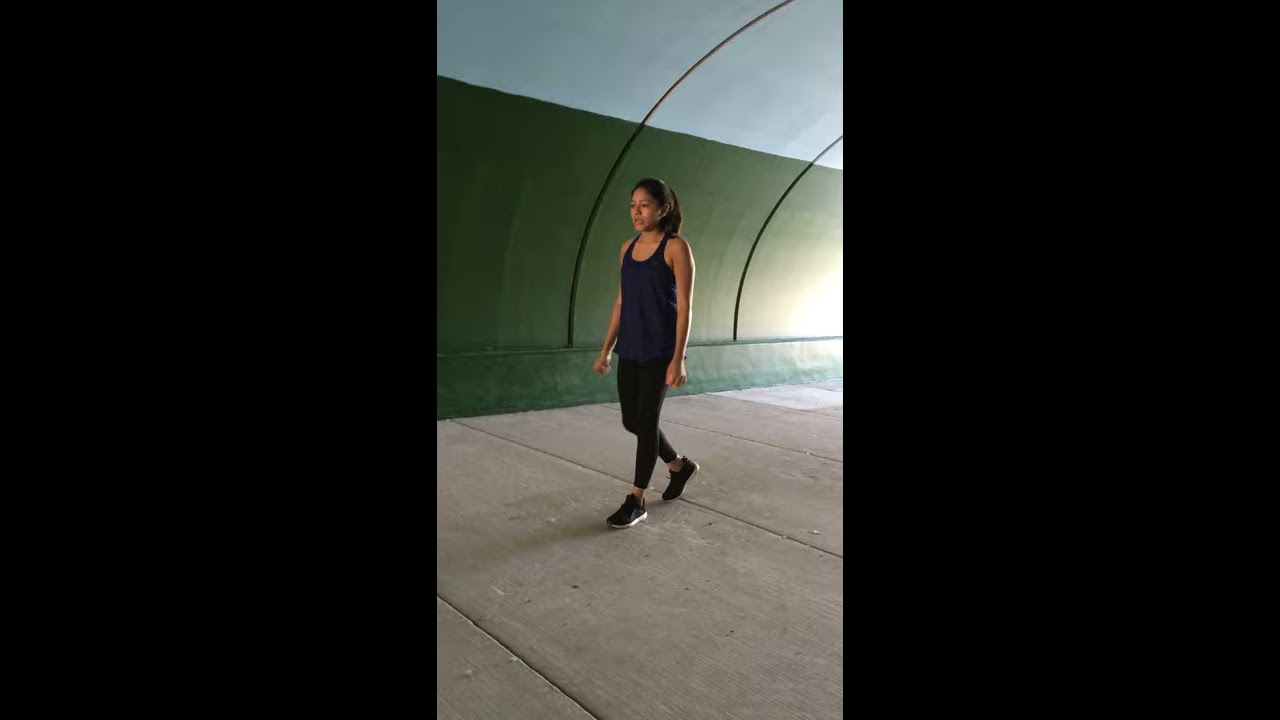In this image, a woman is walking in the center of what appears to be a tunnel or dome-like structure. The tunnel has an arched roof with green stripes running horizontally across it, transitioning to white towards the top, and has two black ribs curving upward. The ground she walks on is a concrete pavement with visible seams. The woman, possibly South Asian or Hispanic, has caramel-colored skin and brown hair tied into a high ponytail. She is dressed in athletic attire, including a dark blue or purple sleeveless tank top, black leggings stopping just above her ankles, and black sneakers with white soles. The setting seems to be outdoors in the middle of the day, and the dominant colors in the image are tan, green, light blue, black, purple, brown, and white. There is no text visible anywhere in the image, and a unique feature includes vertical black bars that run from top to bottom at each end of the frame.